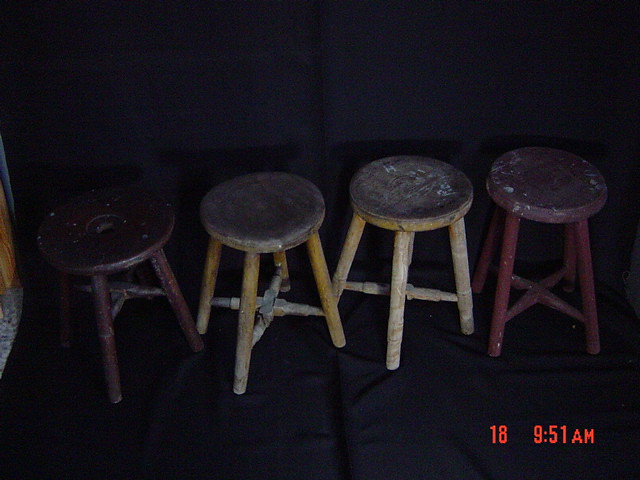In a dimly lit indoor setting, this photograph, timestamped at 9:51 a.m. with the numbers "18 951 a.m." displayed in red at the bottom right corner, showcases four well-worn wooden stools lined up against a wall. The ground beneath them is covered by a black cloth. Each stool is unique in color and condition: the stool on the far left is burgundy with its cross-support placed higher on the legs; the second stool is brown with notable chip marks on its seat; the third stool is light brown, appearing darkest at the top and showing significant wear; and the stool on the far right is red, with its cross-support positioned lower than the others. All stools have round, flat seats, four legs, and a characteristic X-shaped support structure connecting the legs. The stools cast distinct shadows on the wall behind them, and they exhibit signs of extensive use, with paint splatters and a layer of grime adding to their weathered appearance.